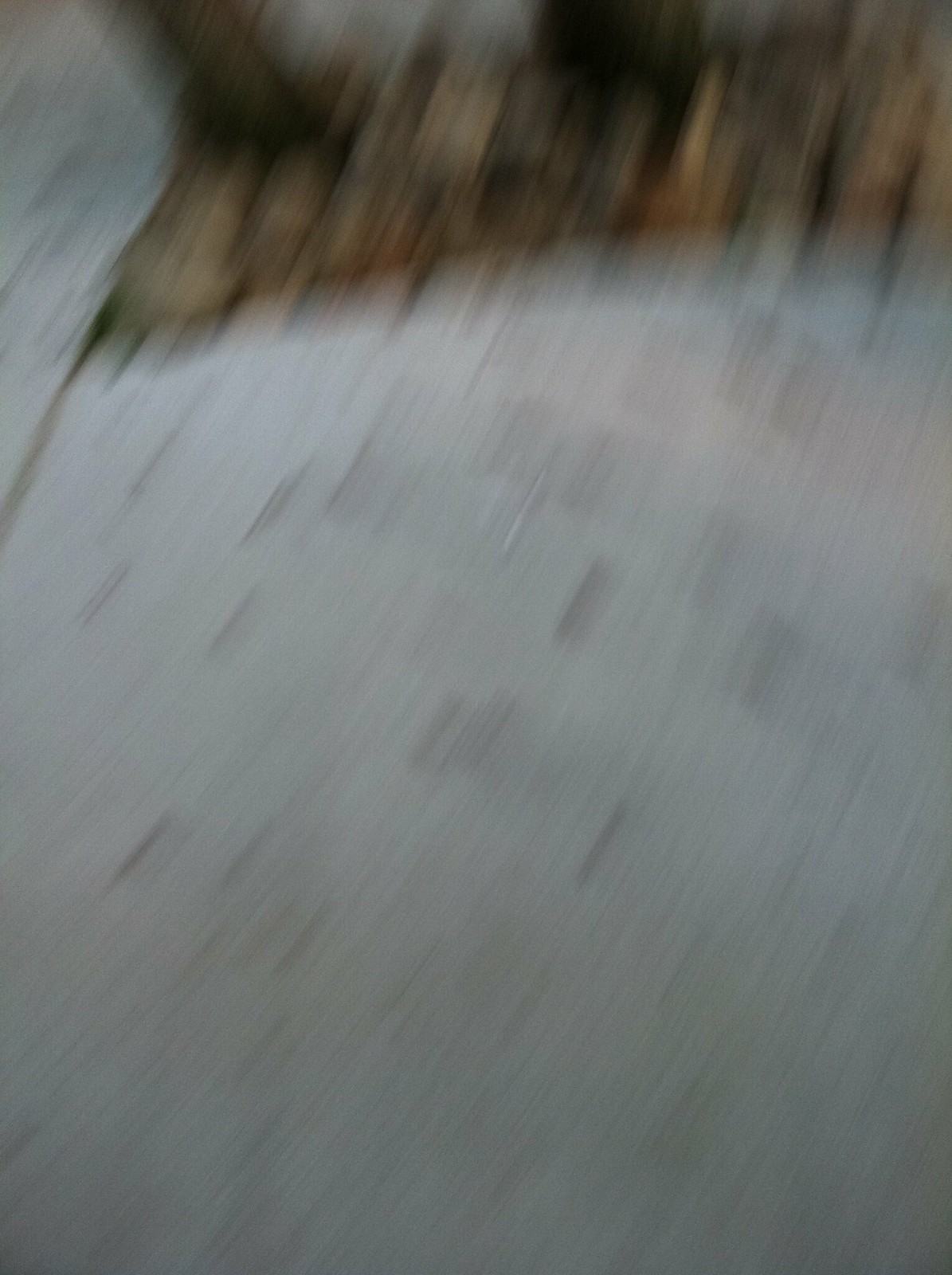The image is a very blurry photograph largely dominated by an off-white and light gray background that occupies around three-quarters of the bottom portion. Diagonal lines in varying shades of gray streak across this area, mimicking brushstrokes. Near the top quarter of the image, the colors shift dramatically to darker tones, featuring heavy lines and irregular, log-like shapes in shades of black, dark brown, and light brown. Some observers suggested it might represent stacked firewood, but due to the extreme blurriness, it’s ultimately ambiguous, teetering between a mere array of brushstrokes and a barely discernible abstract artwork.